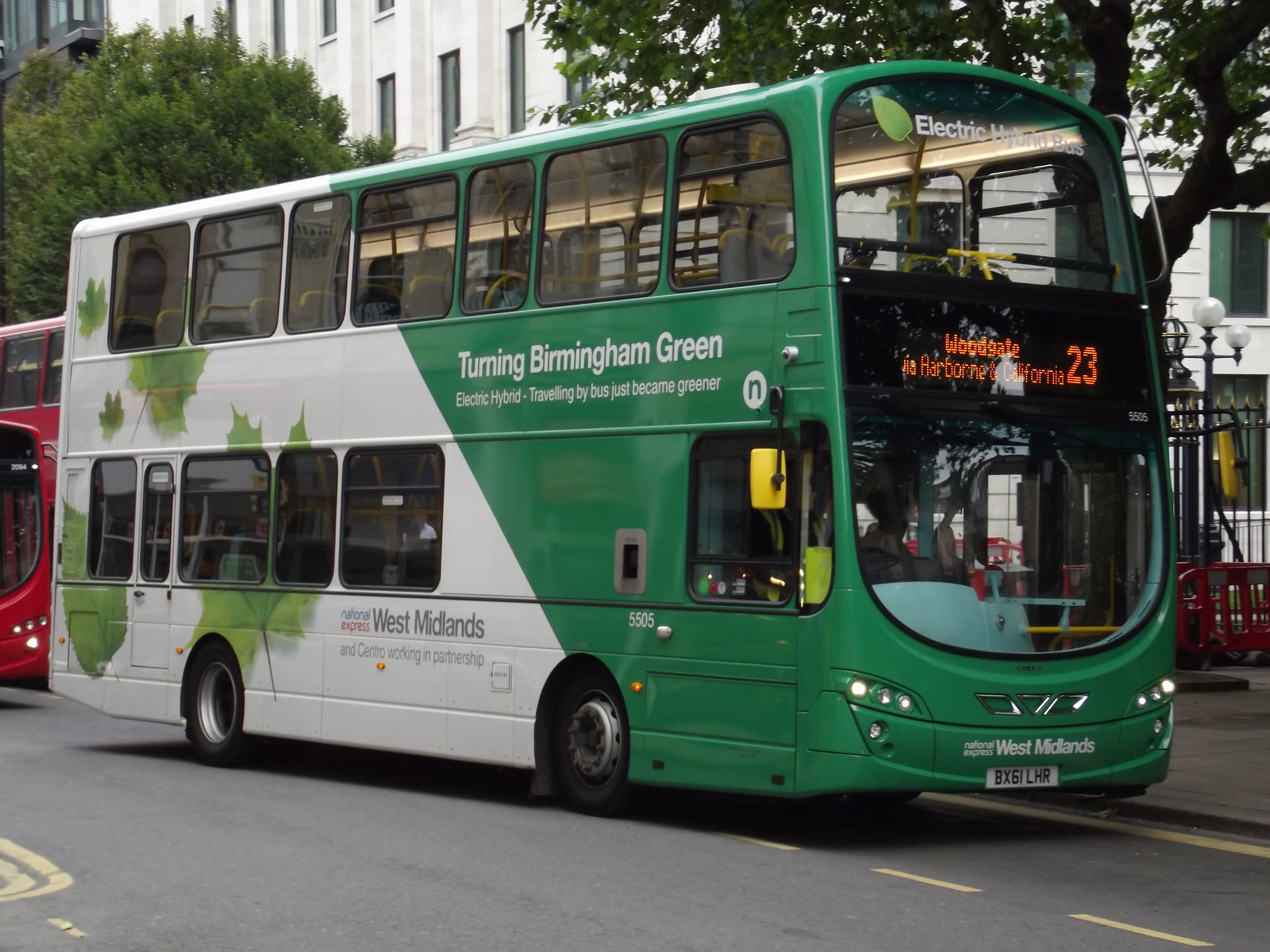This is a detailed photograph of a green and white double-decker bus traveling to the right on a busy city street lined with sidewalks and large green leafy trees. The bus features an advertisement on its side that reads "Turning Birmingham Green" and "Electric Hybrid," emphasizing its eco-friendly nature. The text at the bottom of the advertisement and on the bus itself in black reads "West Midlands." The illuminated sign on the front of the bus displays the route number "23" to "Woodgate" in orange. The upper front windows, where passengers sit on the top deck, also prominently display "Electric Hybrid." The bus is seen passing in front of a large, white building, and while there are no distinct people visible, the shadows of passengers inside can be faintly seen. The scene, likely in Birmingham given the contextual clues, gives off a vibe similar to urban areas but distinct from the traditional London double-decker buses.